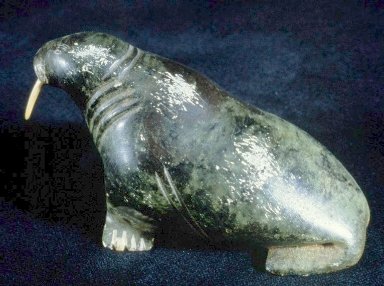The image displays a finely detailed carving of a walrus, resting on a textured blue background that resembles a fibrous carpet or velvet. The walrus, facing towards the upper left portion of the picture, boasts prominent white tusks extending downward from its mouth. The body of the walrus exhibits a dark gray to bluish hue with hints of greenish-gray, suggesting a composition of soft stone or possibly a painted material, though some paint appears scratched off. Intricate chiseled lines mark the walrus's anatomy: four folds around the back of the neck, three on the shoulder area, and two prominent folds behind the left front flipper. The back flippers are tucked under its body, contributing to the lifelike posture. The overall craftsmanship, despite some worn areas, highlights the artisanal effort in depicting the walrus's natural folds and texture.